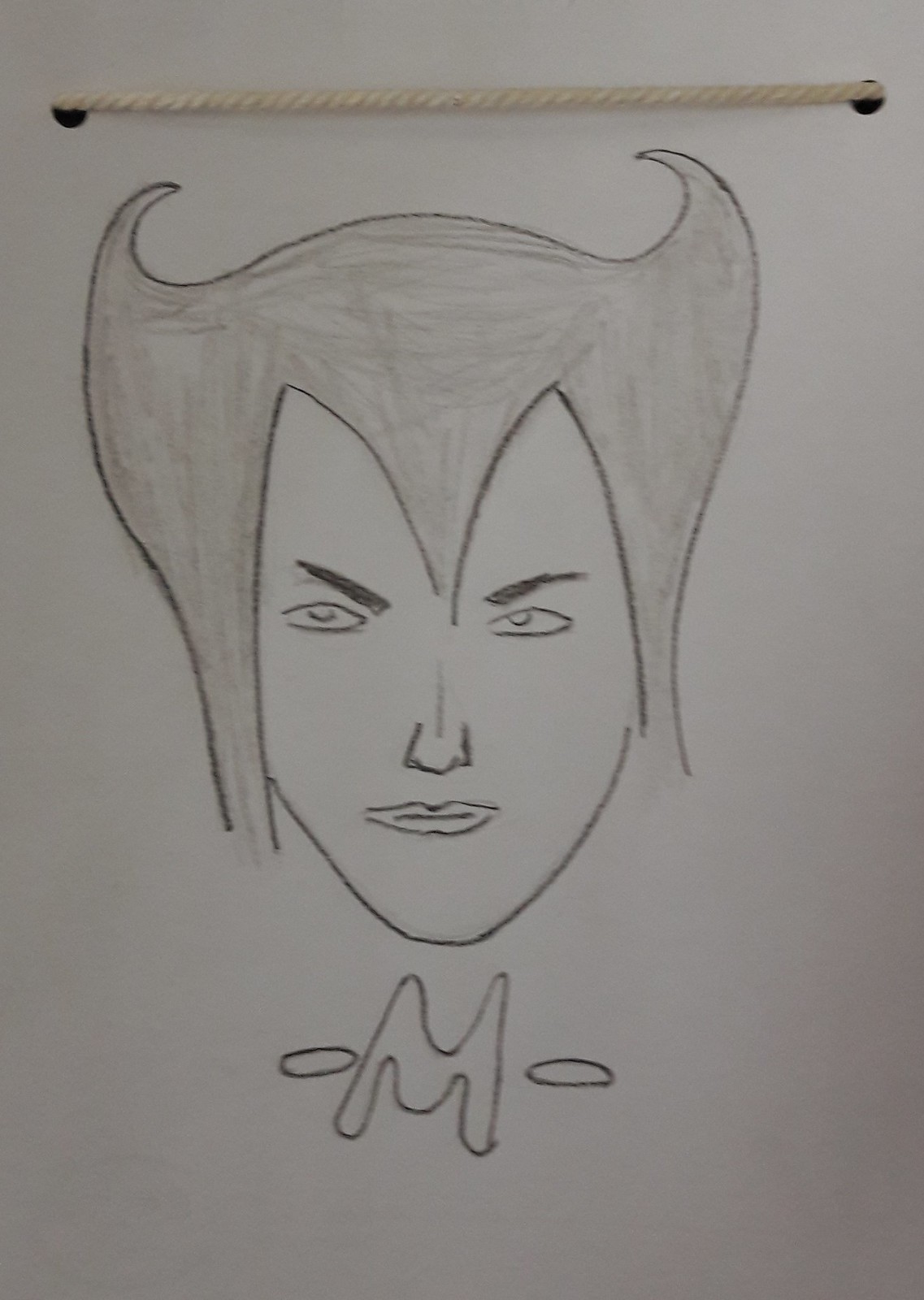The image is a pencil or charcoal sketch on a simple white piece of paper, featuring two holes, punched in the top left and right corners, through which a white piece of string is threaded. This setup suggests that the sketch is meant to be displayed or hung up. The drawing itself is a portrait of a person with distinctive manga-inspired features. The person has hair styled to point down toward the middle of the forehead, almost touching the nose, and flaring out into two horn-like shapes at the temples. The face includes distinct elements such as thin eyebrows, squinted eyes with visible pupils, a small nose with a vertical line extending upward, and lips. Below the face, there is the outline of a capital letter "M," flanked by a horizontal oblong shape on each side. The entire composition, though simple and perhaps amateurish, exudes a unique character and a touch of whimsy.